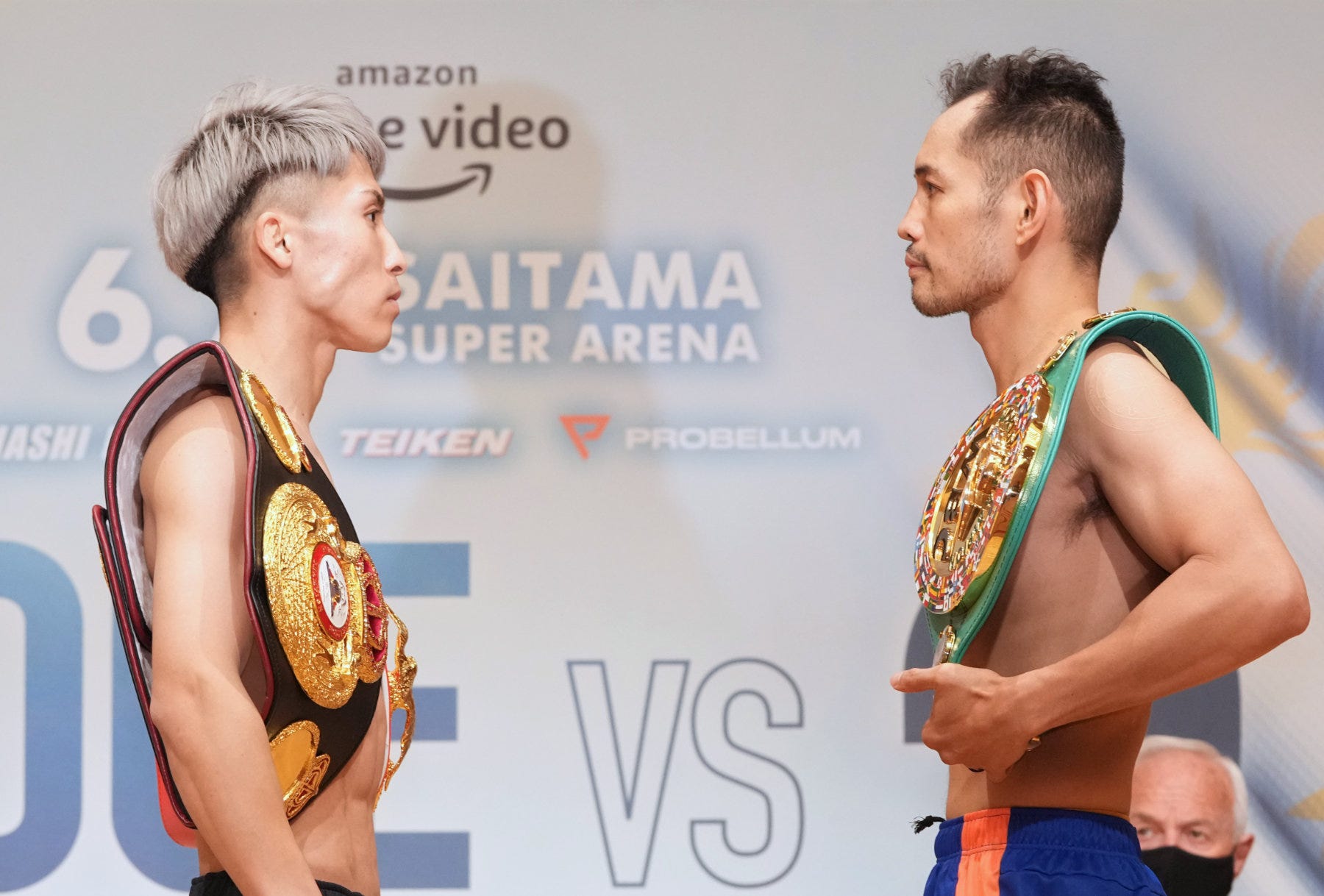The color photograph, likely a video freeze-frame, depicts two determined male wrestlers facing each other. They stand in front of a white banner wall adorned with the Amazon Prime Video logo in black and additional event details in blue. The man on the left, with short platinum-dyed hair that’s black underneath, is shirtless and wears black pants; his black belt features golden rings. He holds a gold championship belt over his shoulder. The man on the right, with short black hair, is also shirtless and dons blue pants with orange stripes. His green belt, embellished with golden emblems, hangs over his shoulder. Both men, identified as boxers Inouye and Donaire, appear fierce and ready for competition.